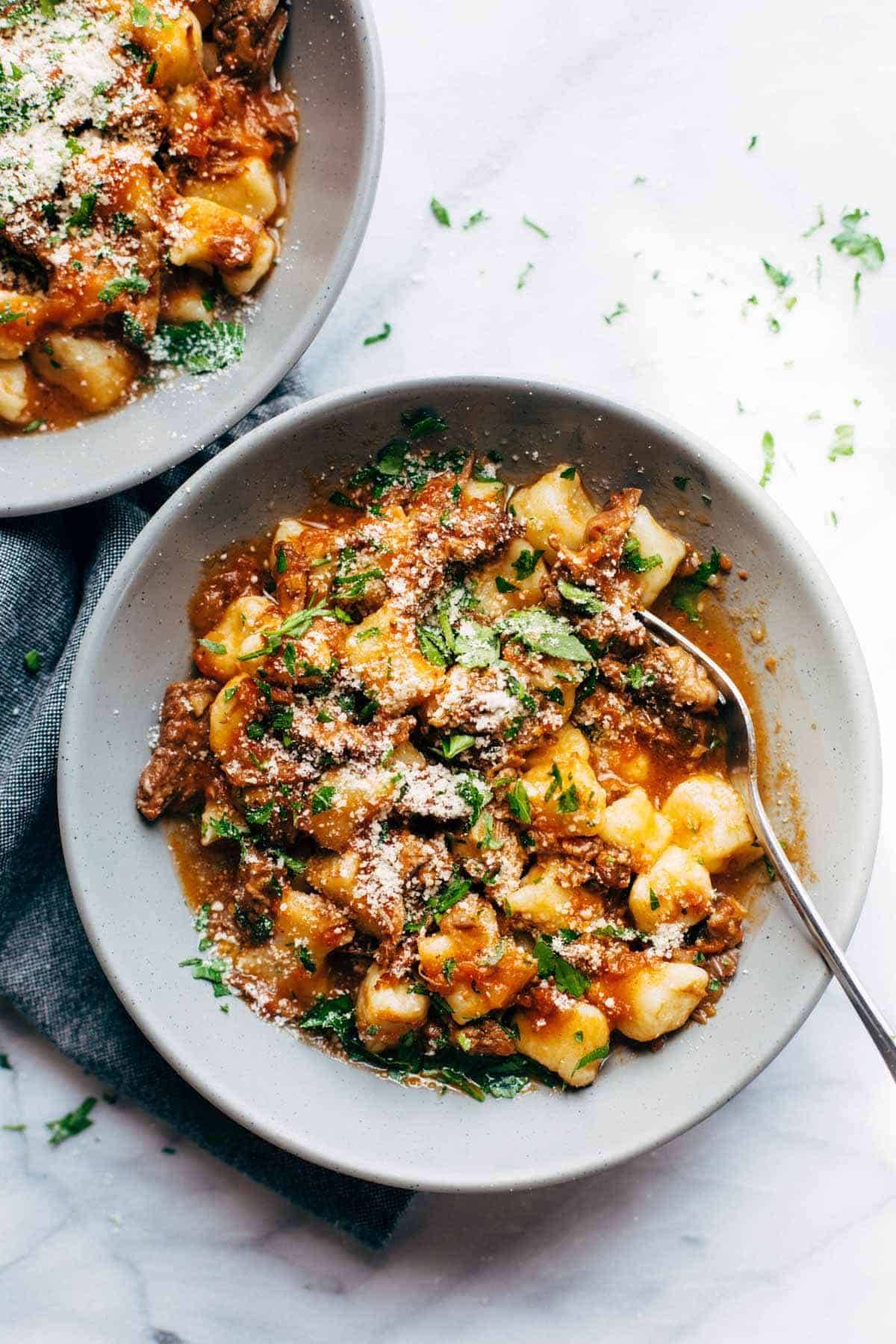The image showcases two servings of gnocchi dishes, each arranged in white bowls, set against a sophisticated white marble table with grey veining. The primary focus is on the bowl in the center, filled with bite-sized dumplings immersed in rich red meat sauce, garnished with chopped parsley and a sprinkling of parmesan cheese. To the right, a fork is partially submerged in the sauce, hanging out of the bowl. Adjacent, in the top left corner, another similar dish appears with a slightly more generous amount of parmesan. The two bowls rest on a dark grey woven cotton rag that adds a rustic touch. In the background, scattered parsley can be spotted on the marble surface, enhancing the overall aesthetic appeal.